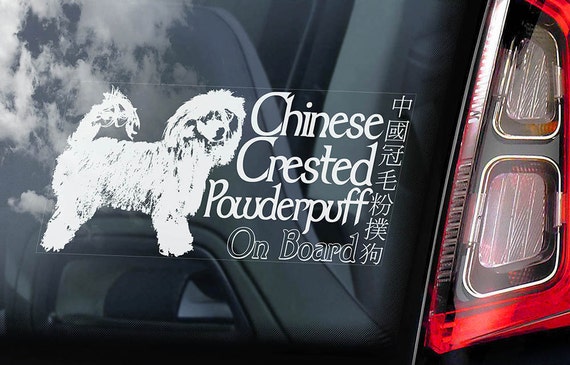This is a realistic photograph featuring the back of a car in a horizontal rectangular orientation. The left section of the image shows dark glass or black metal, reflecting a blue sky with white clouds. On the right side, there are distinct red tail lights with two central white lights, both of which are turned off. A transparent, horizontally-oriented bumper sticker or decal is prominently displayed, likely on the window. This sticker features a detailed white image of a Chinese Crested Powderpuff dog with curly, hairy fur, a fringed tail arched over its back, pointed nose, and long, hairy ears. The dog is depicted in a formal stance, as if being judged, with its front and back legs positioned accordingly. To the right of the dog image, white text reads "Chinese Crested Powderpuff on board," accompanied by a vertical column of Chinese characters.